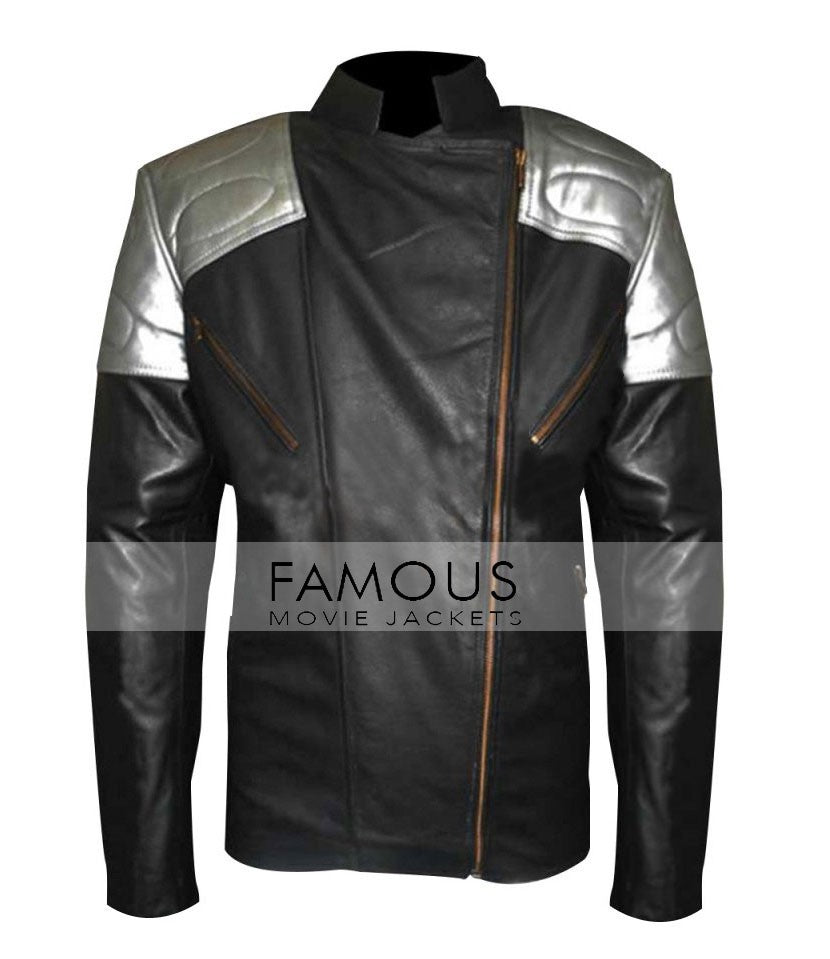The image features a black leather jacket with long sleeves and a distinctive one-inch collar that wraps around the neck. The jacket stands out with its asymmetrical front zipper that runs slightly off-center to the left, leading up to the left shoulder. The zippers, which are a dark, coppery-bronze shade, include two chest pocket zippers that angle from the breast towards the armpits. Adding a unique touch are the metallic silver shoulder pads, complete with quilted oval stitching that extends to the upper arms. A notable feature of the jacket is a translucent white banner across the front, around the belly button area, with bold black lettering that reads "Famous Movie Jackets." The background of the image is white, highlighting the jacket's sophisticated and stylish design.